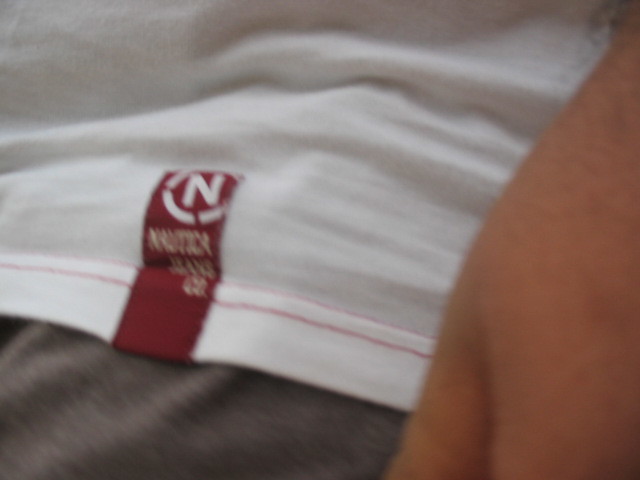The image is a blurry, close-up color snapshot focusing on the tag of a white T-shirt, specifically from the Nautica brand. The person in the photo is pulling down the bottom hem of the T-shirt, revealing the rectangular label that features a red "N" inside a white dashed circle, along with the word "Nautica" and some smaller, unreadable text beneath it. The tag itself is a dark plum color and is sewn onto the hem of the shirt with visible red stitching. The bottom left corner of the photo shows a wavy gray fabric, possibly sweatpants. Along the right-hand side of the image, a hand is partially visible, likely belonging to the person adjusting the shirt. The photo's overall low quality and blurriness make it difficult to discern finer details, but the garment and tag are clearly identifiable.